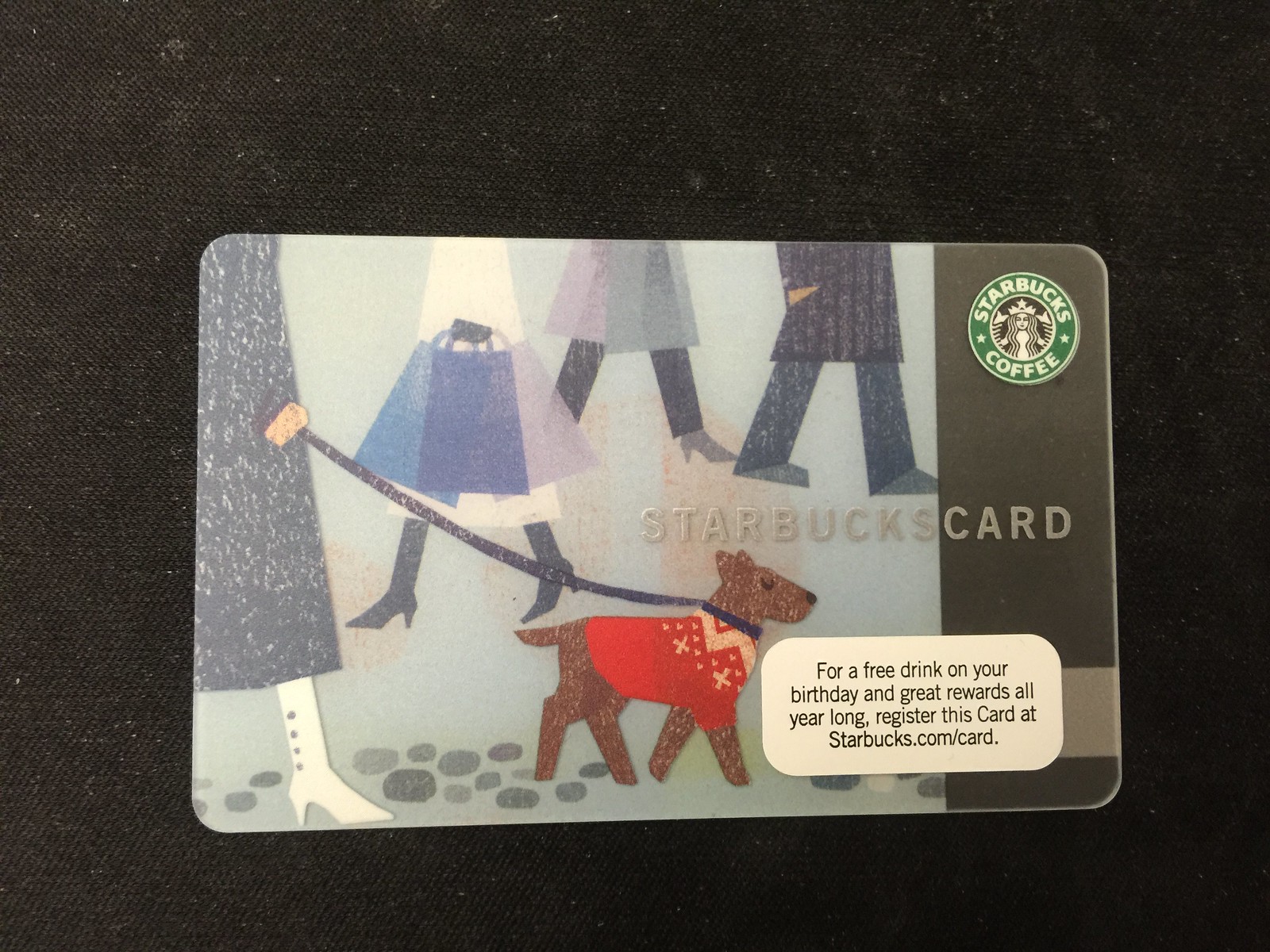The image showcases a photograph of a Starbucks gift card centered on a dark fabric background, possibly denim. The card features an illustration depicting several people walking in the snow from the waist down, accompanied by a small dog wearing a sweater. The dog, with its eyes closed, appears to have a smug expression. On the right side of the card is a vertical brown band, and the left side houses the main illustration. At the top of the card, "Starbucks Card" is prominently displayed along with the Starbucks coffee logo in the upper right corner. Additionally, a white sticker on the card provides information about registering the card online for benefits such as a free drink on your birthday and year-long rewards. The setting suggests the photo was taken indoors. The color palette of the image includes black, gray, light blue, white, red, brown, and green.